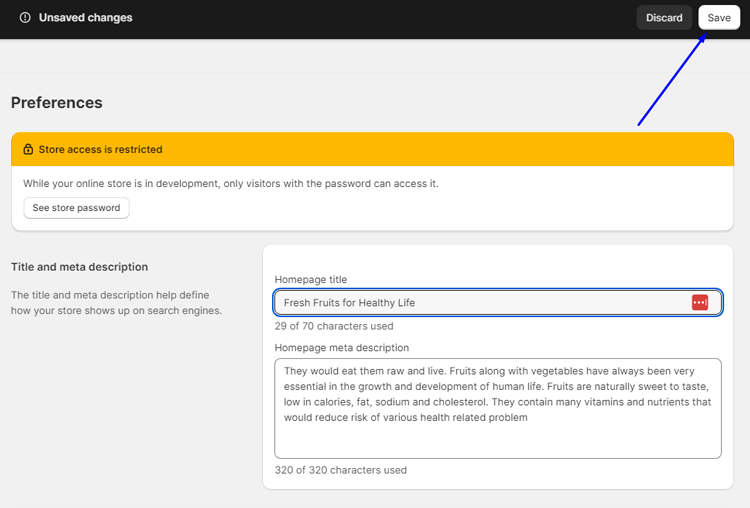In the image, at the very top left corner, there is a label that reads "Unsaved Images." Directly to the top right corner, there is another label that says "Discharge." Next to the "Discharge" label, there is a black-colored box that also says "Discharge," and adjacent to it, there is a white-colored box labeled "Save." A long blue arrow points to the "Save" button, indicating action.

Below this section, the word "Preferences" is visible, followed by a note stating "Store access is restricted. While your online store is developed only visitors with the password can access it." Beneath this note, there is a box labeled "See Store Password" with another blue arrow pointing to the "Save" button.

Further down, there is a heading that reads "Title and Meta Description." This section explains that the title and meta description help define how your store appears on search engines. To the left bottom corner, there is a concise summary of this, while to the right, a large white box labeled "Home Page Title" contains the text "Fresh Fruits for Healthy Life (29 of 70 characters used)." Adjacent to this box is a section labeled "Home Page Meta Description," which contains the following description:

"They would eat them raw and alive. Fruits, along with vegetables, have always been very essential in the growth and development of human life. Fruits are naturally sweet in taste and low in calories, fat, sodium, and cholesterol. They contain many vitamins and nutrients that can reduce the risk of various health-related problems."